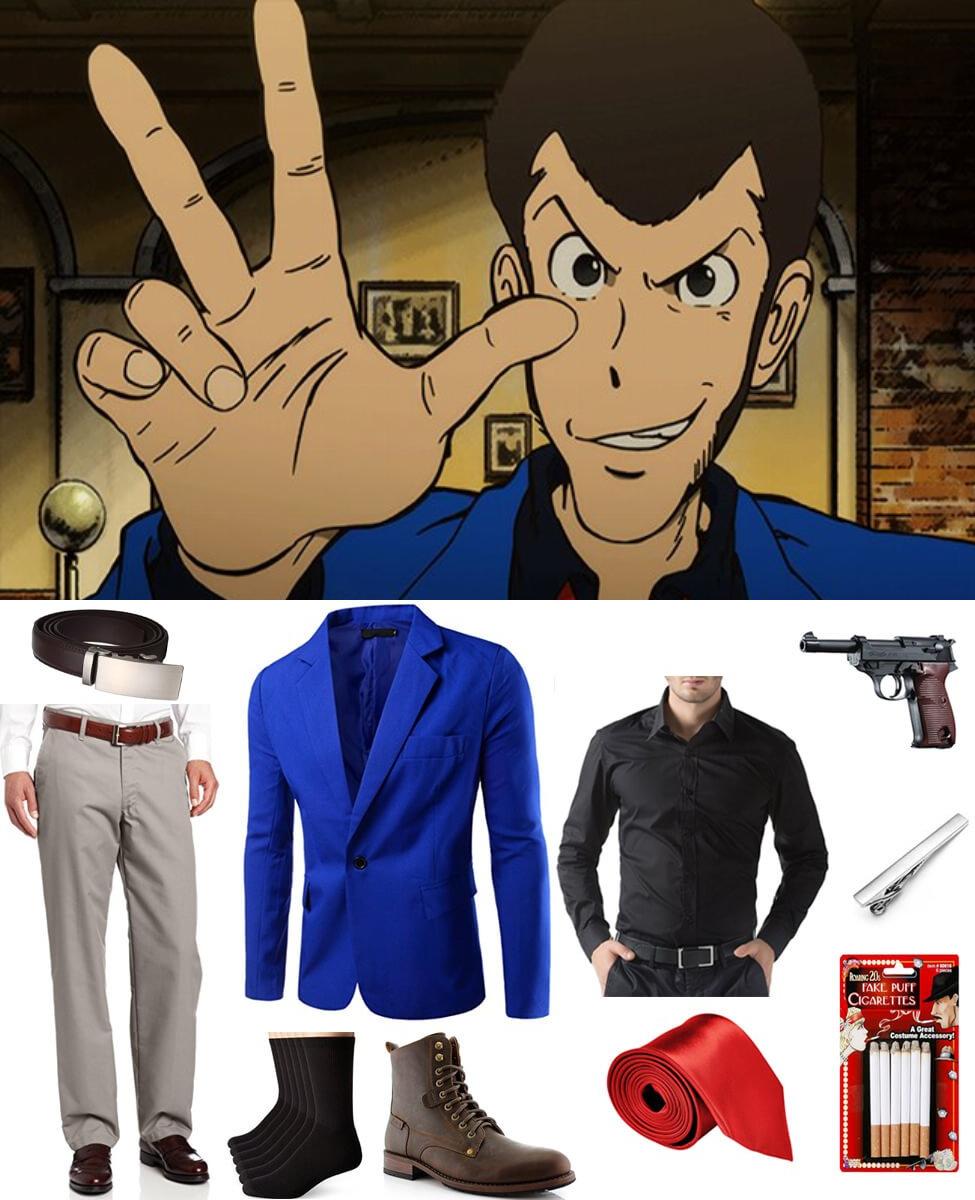The image is divided into two sections. The top half features a cartoon character with a sinister expression. He has short brown hair, dark eyes, and distinctive ears. His hand is raised with the thumb, pointer finger, and middle finger extended, while the other two fingers are folded down, as if signaling the number three. He wears a dark blue blazer over a black undershirt and stands against a beige and light brown wall with orange accents and framed pictures. A red, pink, and gray brick wall is visible to the right.

The bottom half of the image showcases various outfits and accessories that match the character's attire. This includes a dark blue blazer with a black button and a V-neck shape, black socks, and brown boots with brass rivets. Also featured are a man’s torso with light skin wearing gray trousers, black or dark brown shoes, a white undershirt, and a black belt with a silver clasp. Additional items include a long-sleeved black shirt paired with black pants and a similar belt. A red silk tie is rolled up next to a black-brushed metal Ruger pistol with a wooden handle, an unidentified metal object, and a sealed container of fake puff cigarettes.

The detailed clothes and accessories in the bottom half strongly resemble those worn by the character in the top half, connecting the animated figure to the real-world items below.